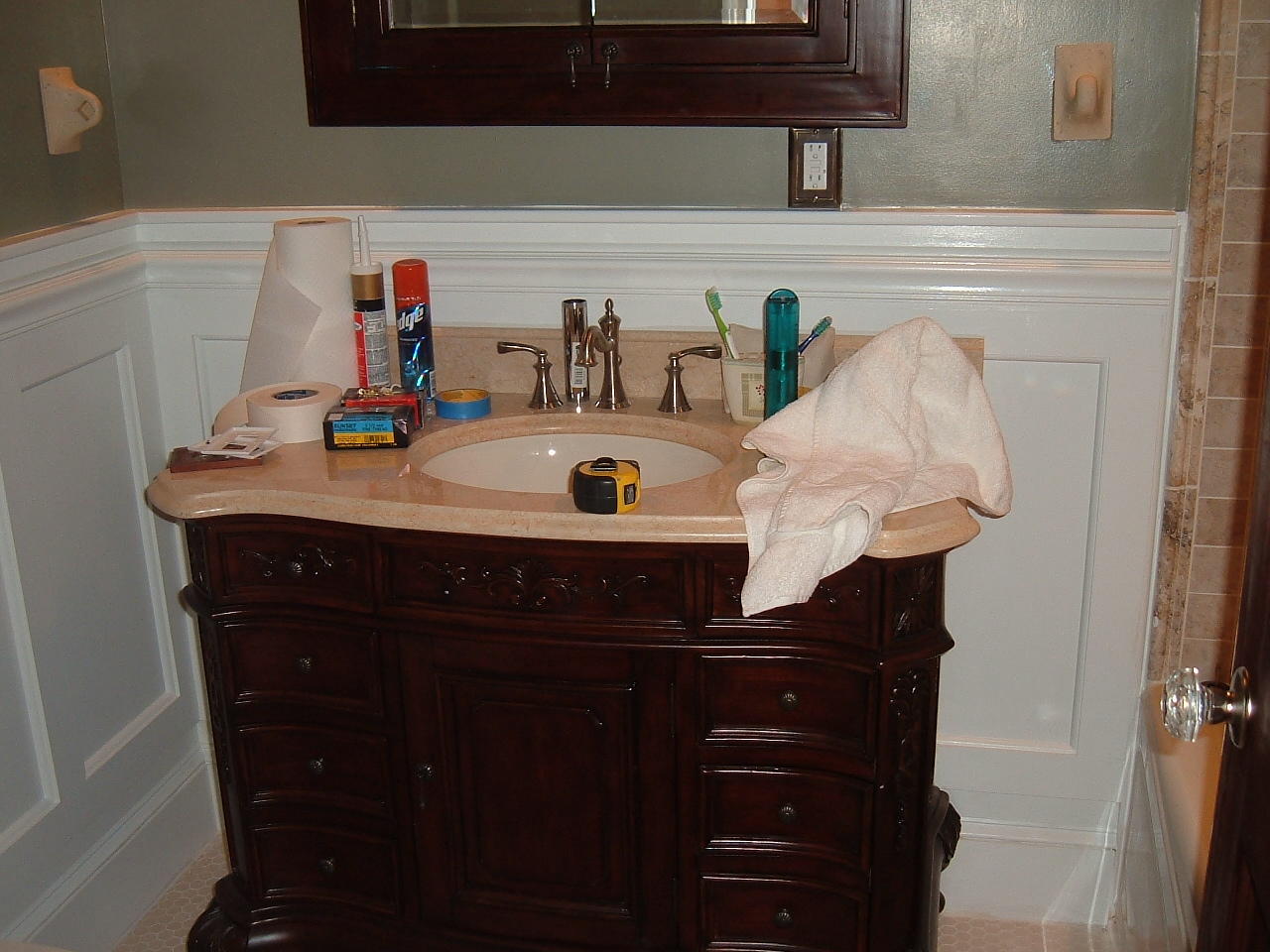The photograph captures a detailed view of a bathroom sink area. The countertop is made from beige-colored marble, accentuating a white circular sink basin equipped with a silver faucet and two lever-style handles on either side. The front of the countertop boasts dark wood cabinetry, with almost black drawers and a central cabinet door. The background features white wooden paneling on the lower half of the wall and a grayish-green paint on the upper half. On the far right of the image, a glimpse of a beige-tiled shower or bathtub is noticeable along with the edge of a door that matches the dark cabinetry, featuring a metal and clear crystal door handle in the lower right corner.

A dark-edged mirror hangs above the sink, reflecting the cohesive dark wood theme. The sink area is cluttered with various items: a yellow and black retractable measuring tape lies in front of the sink, a crumpled white bath towel occupies space on the right side, and a roll of paper towels is positioned in the back left corner. Nearby, a roll of tape, several cans of cleaning solution, a box that likely contains screws or nails, and several white plastic panels designed for covering light switches or power outlets rest on the counter. Additionally, a cup holding two toothbrushes is situated to the right of the sink, completing the scene.